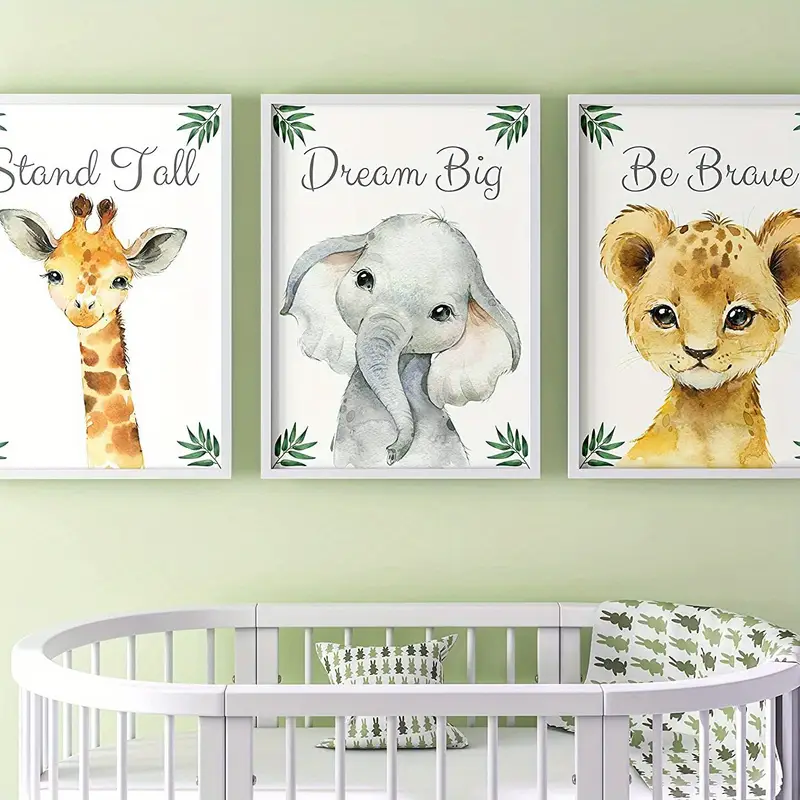This image appears to be an advertisement for a nursery, showcasing an adorable and well-decorated nursery room. The focal point is an oval, white crib with a white mattress, complimented by a blanket and pillow adorned with patterns of dark and light green bunny silhouettes. The crib sits beneath a mint green wall, which is home to three large, white-framed pictures. Each picture features a watercolor baby animal with big, expressive eyes set against a white background with green leaves in the corners. The left picture displays a sweet giraffe with tan and brown features, gray ears, and little brown horns, accompanied by the motivational phrase "Stand Tall" in gray cursive. The center picture shows an adorable gray elephant with large ears and a playful demeanor, under the words "Dream Big". The right picture captures a tan and brown-spotted cheetah with a friendly expression, captioned with "Be Brave". Together, these elements create an inviting and whimsical nursery space.